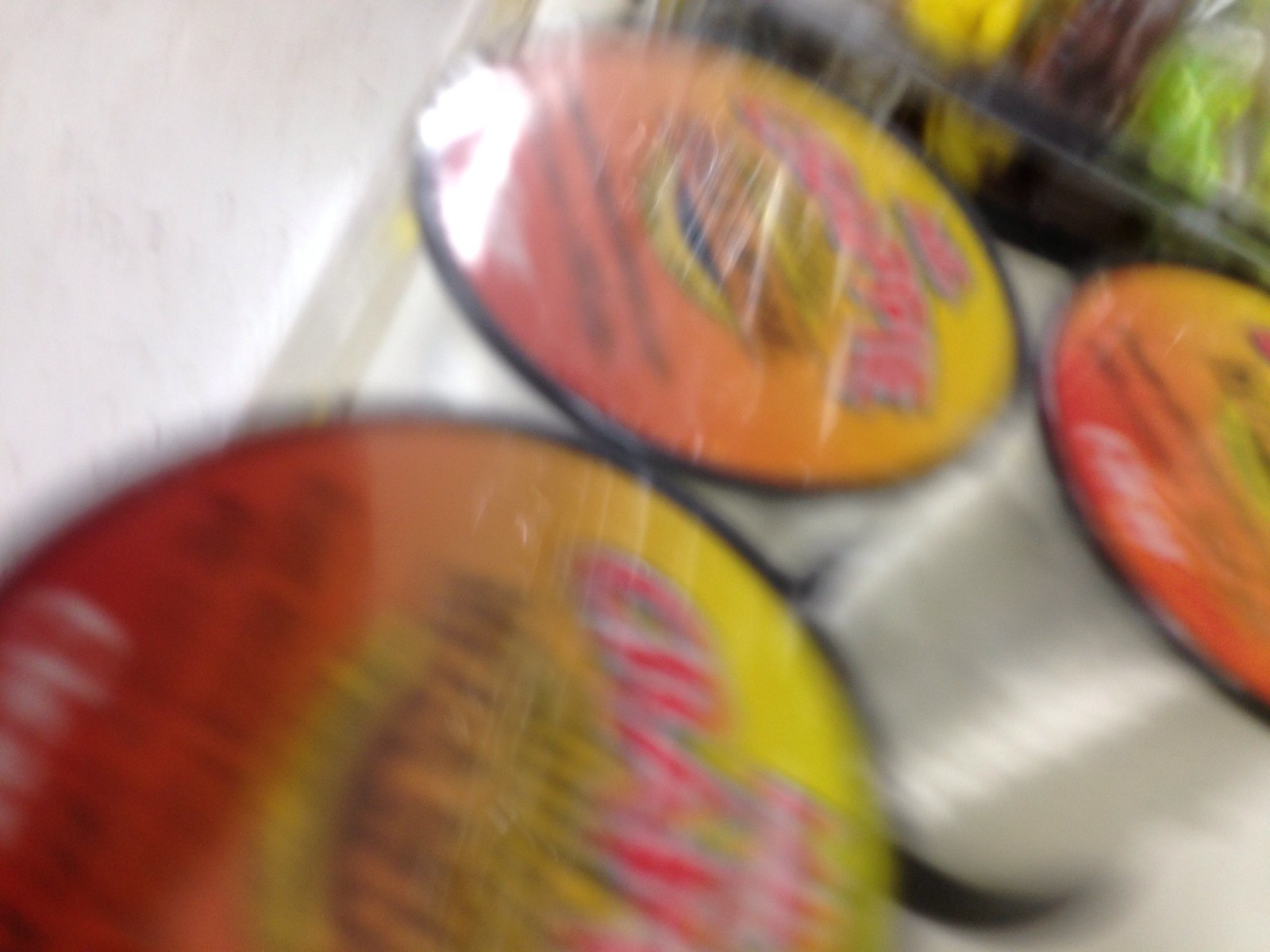The blurred colour photograph showcases a trio of cylindrical items, likely products in a store setting. The image is taken at a skewed angle, necessitating a 90-degree clockwise rotation to properly view it. Each cylindrical object features a yellow top transitioning to orange and then red towards the bottom, with red text on the yellow top. The items exhibit a reflective white surface with streaks of light and black borders at both the top and the bottom. The cylindrical objects are partially encased in cellophane, suggesting they are some form of packaged goods, potentially ramen or spools of string/twine. Three of these identical items dominate the foreground, with two prominently side-by-side and one slightly set apart. Additional elements like a green vegetable or fruit and possibly other items, including something purple, are visible but indistinct due to the image's blurriness. A white wall or barrier occupies the upper left corner, contributing to the overall impression of a cluttered store shelf.